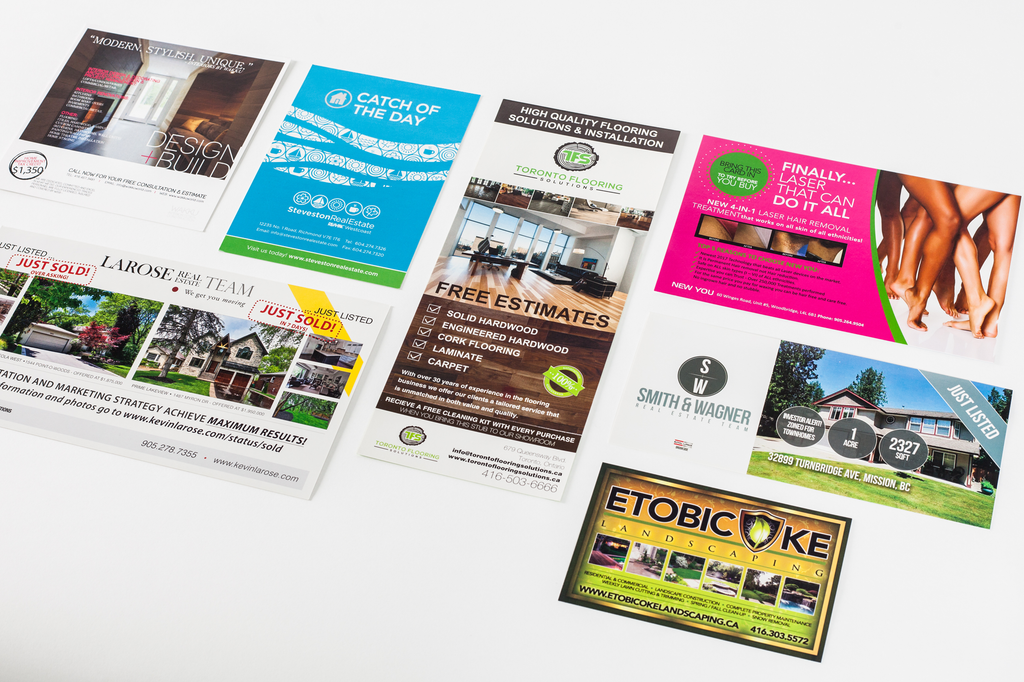This photograph showcases a collection of seven rectangular flyers and pamphlets arranged on a white floor, each advertising various local businesses and services. The flyers come in a variety of colors – white, blue, pink, brown, and green – and each features promotional text. The top left flyer reads "Modern Stylish Unique Design + Build" and includes a partially visible dollar sign with "1350." The next flyer, primarily blue, advertises a local restaurant with the text "Catch of the Day" and mentions "Steveston Real Estate." There's a flooring service flyer proclaiming "High Quality Flooring Solutions and Installation Toronto," detailing different types of flooring and offering free estimates, as well as a free cleaning kit with every purchase. The bottom left flyer from "La Rose Real Estate Team" highlights properties just listed and successfully sold, including banners like "Just Sold Over Asking" and "Just Sold in Seven Days." The top right flyer, in bright pink with green accents, promotes a "4-in-1 Laser Hair Removal" treatment for all ethnicities, with an offer to "Try Before You Buy." Additionally, there's an advertisement for "Smith & Wagner Real Estate Team," showcasing a two-story house and an investor alert for townhomes. The final flyer pertains to "ETOBICOKE Landscaping" with several photographs of landscaping projects, providing a contact number and website. Each flyer is distinct yet collectively creates a vibrant display of local business promotions and advertisements.